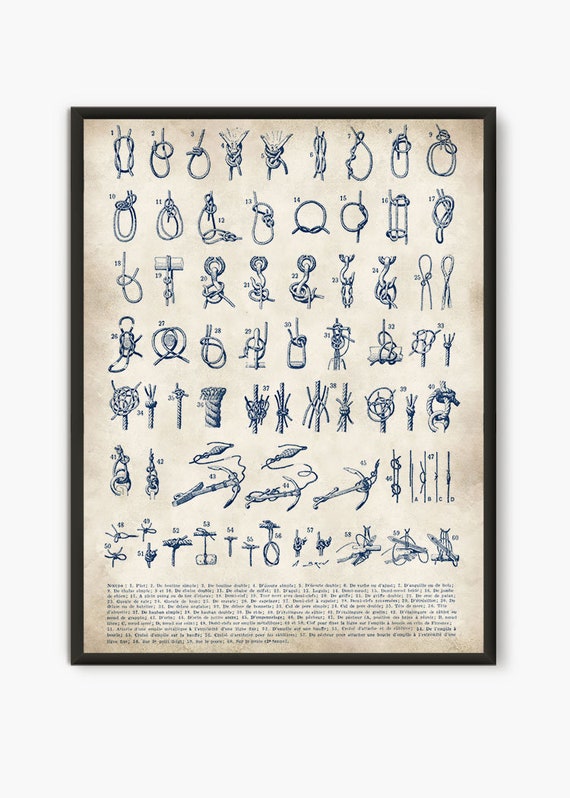This vertical rectangular image features an old, weathered cream-beige background with a black frame. It contains a meticulously arranged collection of around 50 to 60 diagrams depicting various knots and possibly other small figures or tools. Each illustration is numbered, starting with simple knots progressing to more complex ones. The detailed drawings, rendered in navy blue ink, are arranged in neat rows, and the text accompanying them is so small it's almost illegible. Toward the bottom, there is an intricate figure resembling an anchor, along with numerous tiny diagrams and lines, possibly illustrating different stitches or steps. The overall appearance of the paper and the style of the drawings suggest that this is an antique instructional chart or guide.